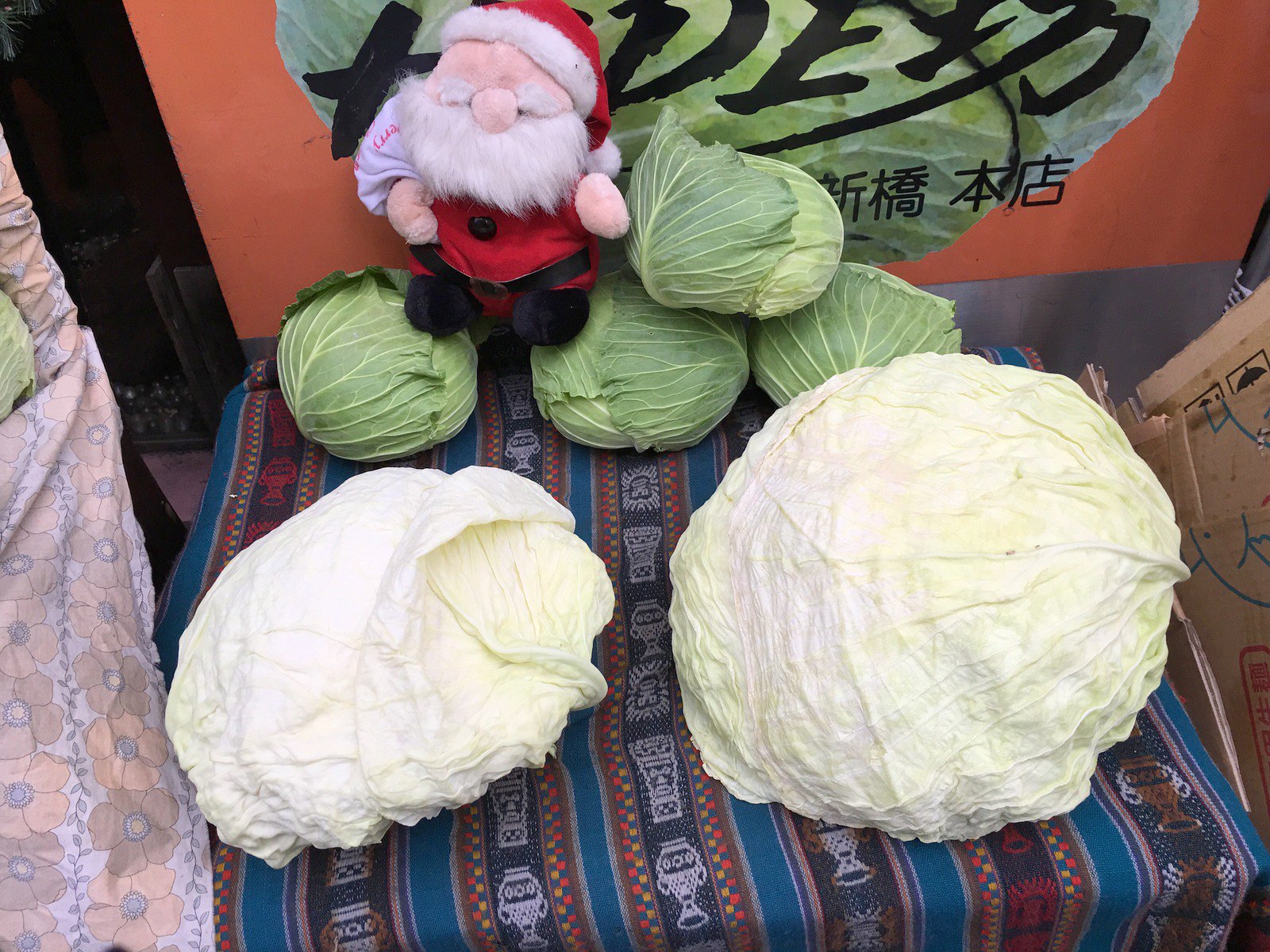The color photograph depicts a detailed scene centered around various cabbages arranged on a stool draped with a turquoise and white striped cloth featuring gray embroidered designs of vases and urns. In the foreground, there are two large, light-colored, tightly-headed cabbages, resembling Napa cabbage in color but more compact in shape. Behind these, three smaller green heads of cabbage are positioned horizontally, with a fourth green head perched on top of the right two. Adding a festive touch, a small plush Santa Claus sits atop the left and center smaller heads.

In the background, a square orange-framed sign or glass panel with a translucent middle surface can be seen. This panel bears black writing in Japanese or Chinese characters, along with some partially visible English text. The translucent part appears to depict or reveal cabbages behind it, enhancing the thematic consistency of the image.

To the right of the stool is a cardboard box, and a floral-covered chair is partially visible to the left, contributing to the scene’s cozy, eclectic feel. The entire image is in sharp focus, bringing out the intricate details and textures of both the cabbages and the surrounding elements.